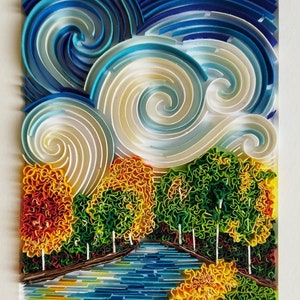This small, square digital image showcases an intricate art piece resembling a mosaic or a mosaic-like illustration, perhaps incorporating materials like macaroni or different noodles. At the bottom of the image, there's a blue, paved walkway, almost glass-like, lined with a mix of a yellow and green bush. This path is flanked by tall, slender trees with autumn foliage, displaying an array of colors from red and yellow on the left to predominantly green on the right. Above the trees, the sky is filled with large, shiny swirls in white and blue, reminiscent of the swirling patterns in Van Gogh's "Starry Night." The entire composition is rich with color and lined details, creating a vibrant and dimensional scene that appears to pop off the canvas. The left and right sides of the image feature beige bars, adding to the layered, three-dimensional effect of the artwork.